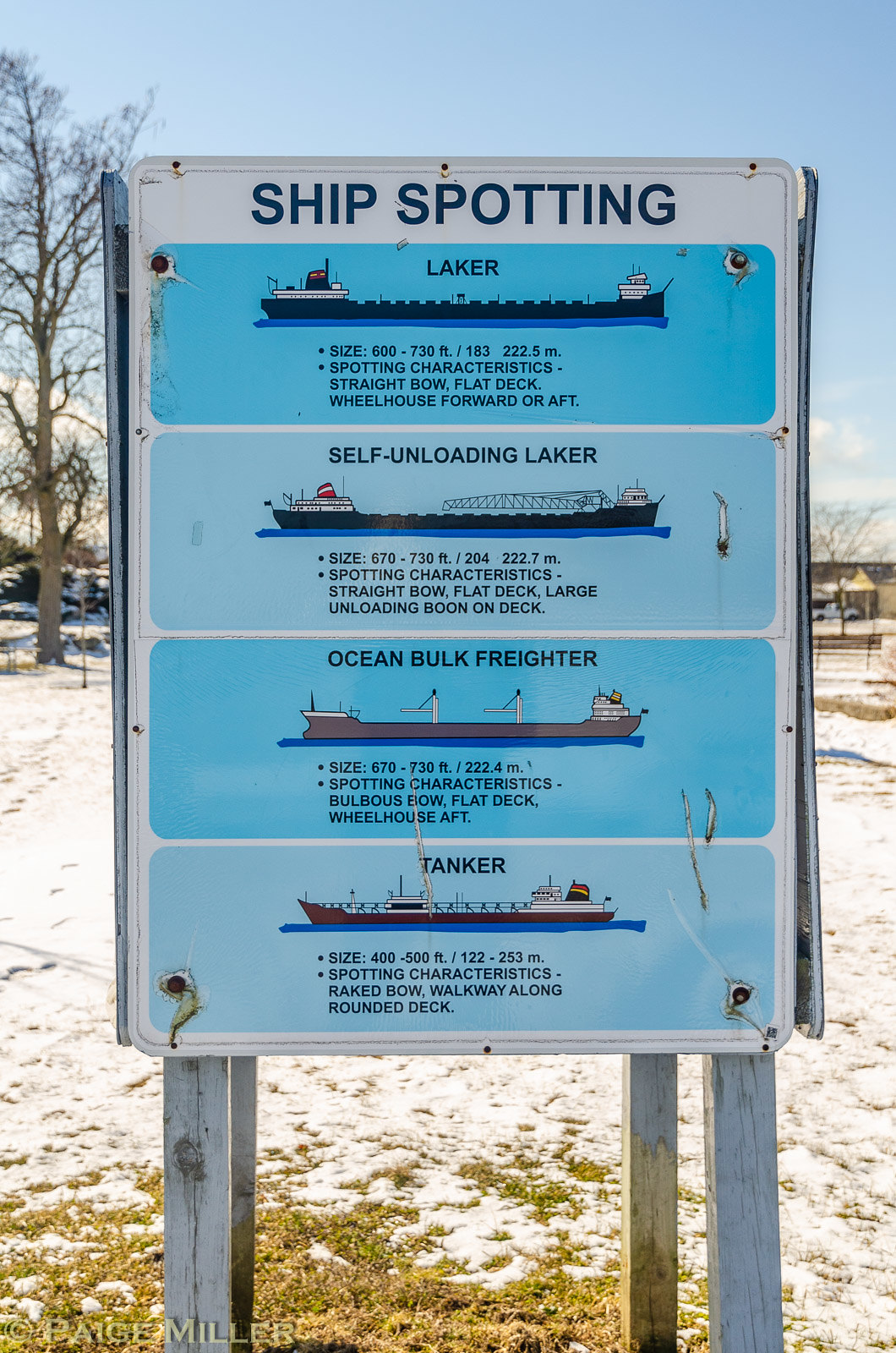This photograph captures an old, weathered sign titled "Ship Spotting," prominently displayed in the middle of a snowy, grassy field, suggesting a winter setting possibly near the Great Lakes. The sign, colored blue and white with peeling paint and noticeable scratches, is supported by four wooden posts, with additional signs possibly flanking it to the left and right. The background features barren trees and a distant structure with a vehicle, grounding the scene further.

The sign details four types of ships, displayed in blue sections with white borders. The first is a "Laker," a long cargo vessel characterized by a straight bow, flat deck, and wheelhouse either at the forward or aft, measuring between 600 and 730 feet. Below it is the "Self-Unloading Laker," similar in size (670 to 730 feet) but distinguished by a large unloading boom on its deck. The third vessel type is the "Ocean Bulk Freighter," featuring a bulbous bow, flat deck, and aft wheelhouse, with dimensions ranging from 670 to 730 feet. Finally, the "Tanker," measuring 400 to 500 feet, stands out with its raked bow and a walkway along the rounded deck. Despite some text being difficult to read due to its small size, the sign remains legible and provides insightful spotting characteristics for each ship type. The ground around the wooden posts shows what might be seaweed, adding to the maritime theme and reinforcing the possibility of its lakeside location.